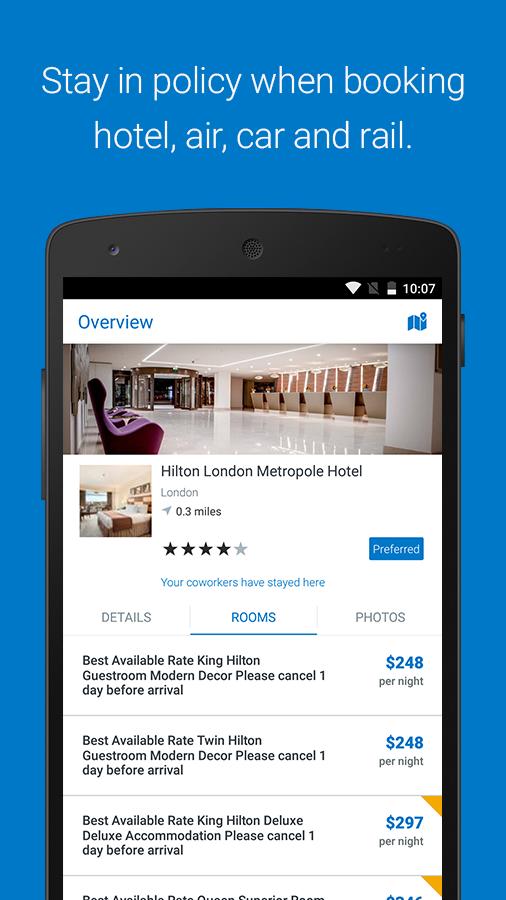**Caption:**

The advertisement, likely sourced from a web page or app store, features a sophisticated design set against a dark blue background. At the top, a bold white text reads, “Stay in policy when booking hotel, air, car, and rail.” Below, a realistic mock-up of a smartphone with a black bezel and a circular speaker showcases a web page.

The web page begins with a blue header labeled "Overview." A map with a pin and a logo appears on the right side, while on the left side, there is an illustration of a waiting area featuring seats in maroon or violet on one side and white on the other. The interiors include reflective white marble flooring, a predominantly white ceiling and walls, with occasional brown accents.

Beneath this overview, bold text announces “Hilton London Metropole Hotel,” likely the location depicted above. On the left, a bedroom is shown with round and tan sheets, white pillows, and a view outside. The hotel is noted to be 0.3 miles away, with a rating of 4 out of 5 stars. A dark blue rectangle with thin white text indicating "Preferred" accompanies these details.

In the center, clickable blue text reads, "Your co-workers have stayed here."

Three tabs are visible: "Details" in gray, the selected "Rooms" in bold blue with an underline, and "Photos" in gray. The "Rooms" tab provides a list of available options:

1. **King Hilton Guest Room:** Modern decor, requires cancellation one day before arrival, priced at $248 per night.
2. **Twin Hilton Guest Room:** Modern decor, requires cancellation one day before arrival, priced at $248 per night.
3. **King Hilton Deluxe:** Deluxe accommodation, requires cancellation one day before arrival, priced at $297 per night.
4. (Cut off entry).

Each listing's price is displayed in blue on the right side, emphasizing affordability and transparency in booking.